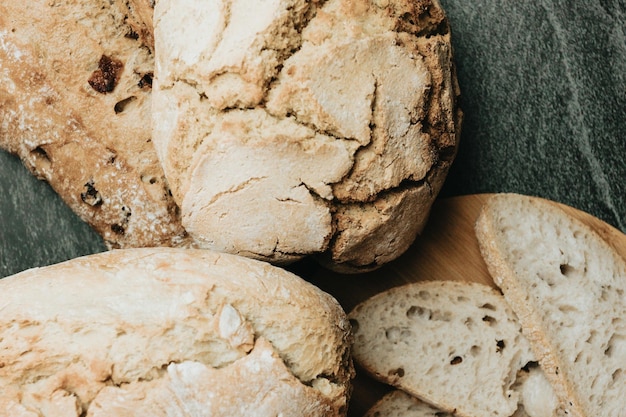This close-up photograph showcases three unsliced, rustic loaves of bread, artfully arranged on a slate dark grey countertop that features mottled coloring with hints of dark green and white streaks. The crusty loaves, distinguished by their deep cracks, are positioned with one to the left, another at a 90-degree angle, and the third nestled between them, slightly overlapping. On the bottom left, a round wooden cutting board holds three thin slices of white bread. Flour dusts the loaves, enhancing the handmade aesthetic, and a variety of textures suggest some might include raisins. The intricate details and arrangement of the bread make this image ideal for a cookbook or a baking class advertisement.